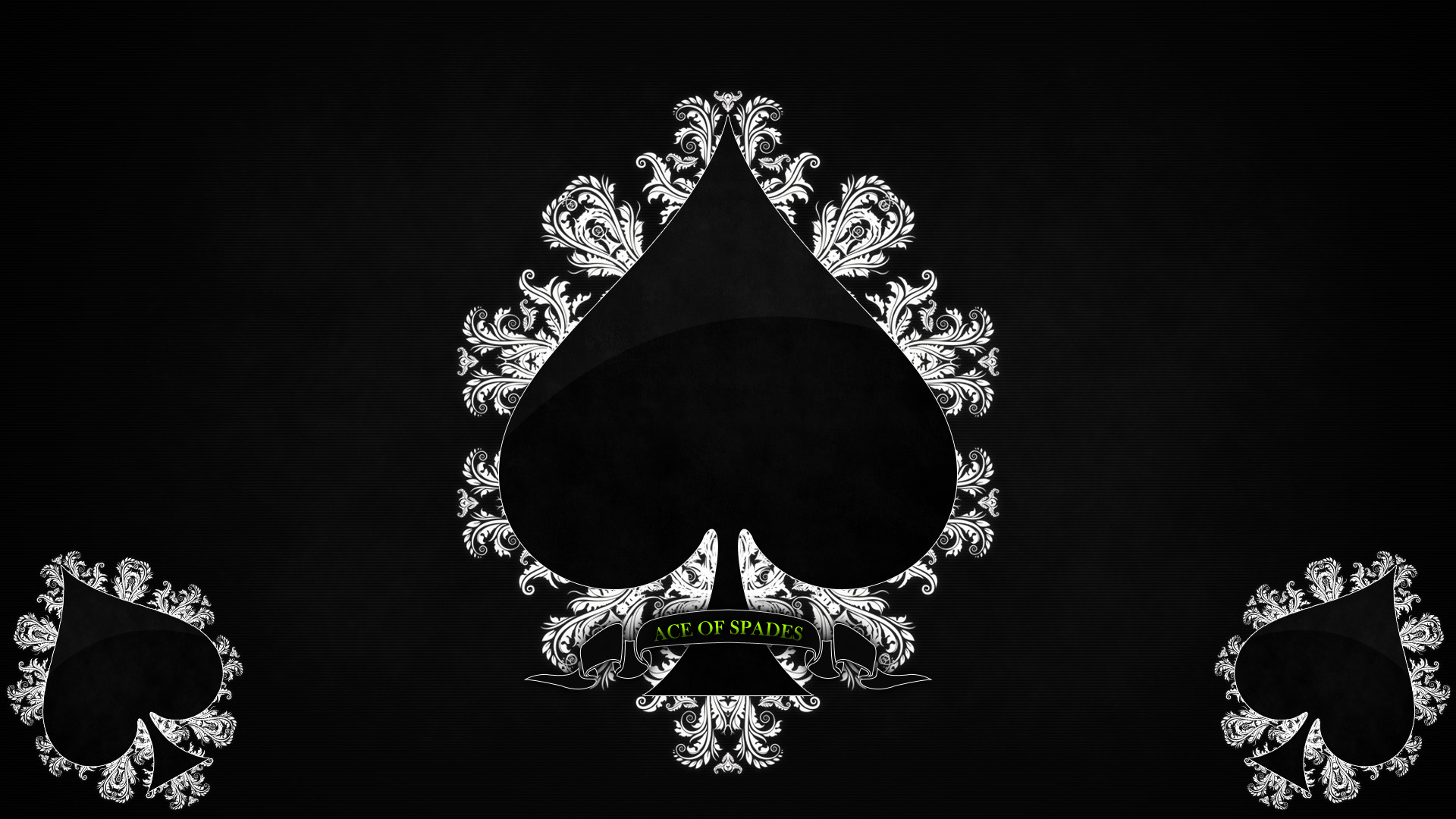The image features a prominently detailed ace of spades card set against a solid jet black background, making the ornate design elements strikingly visible. At the center of the card is a large black spade, resembling an upside-down heart with a stem, identified as the ace of spades by the green capital letters inscribed at its stem. This central spade is enveloped by an intricate white floral pattern that gives a sense of elegance and intricacy to the design. Additionally, two smaller black spades are positioned in the left and right bottom corners, each encircled by the same white floral pattern, echoing the central spade's motif. The symmetry and detailed embroidery create a visually captivating contrast against the dark background, emphasizing the delicate white patterns and the distinct green lettering within the spade's design.